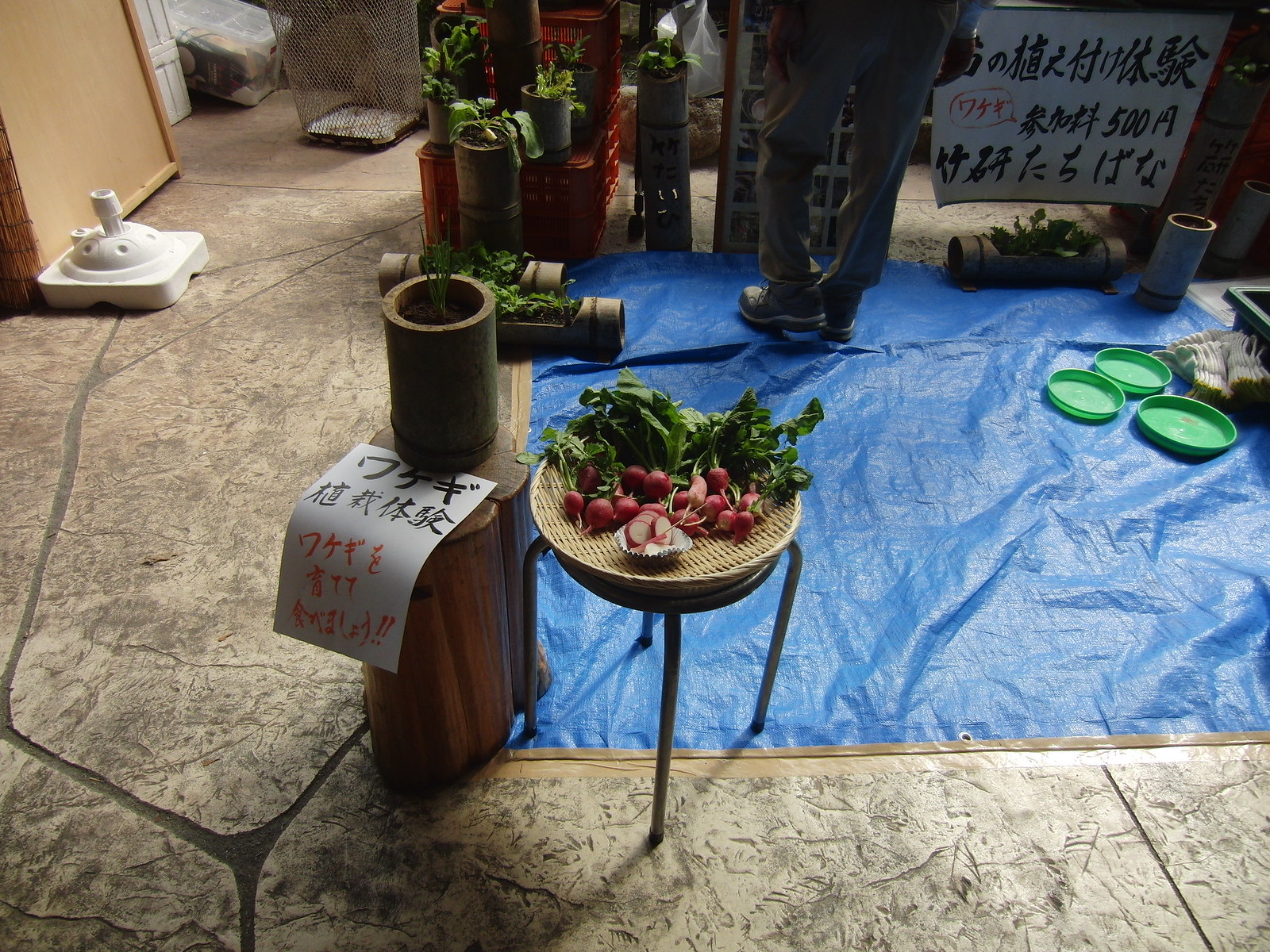This photograph captures the scene of what appears to be an indoor farmer's market with an eclectic mix of items and vibrant cultural elements. The setting resembles a living room but has the feel of an outdoor market due to the various signs and setup. Dominated by a blue tarp laid out on the hard floor, the market features several key items and decor elements. In the center, there's a small four-legged coffee table stand with a wicker basket holding a bunch of red, pinkish radishes, some of which are cut up in a little white bowl. Surrounding the radishes, various containers and baskets are strewn about, including green bowls and cylindrical wooden planters with green spices or plants growing out of them.

To the left, hanging off a greenish fake stump, is a sign with black and red Chinese or Japanese writing, denoting another seller's offerings. The top right of the tarp has additional planters and more signs with black ink and red speech bubbles. Above these, another large sign in Chinese or Japanese letters stands prominently. Additionally, red milk crates are stacked, potentially holding more spices or plants.

In the foreground, the lower half of a man in gray slippers and tan pants is visible, seemingly engrossed in the items or signs in front of him. Beyond the market area, the light brown walls and a white door frame the scene. The space feels like a blend of domestic and commercial, enriched with cultural nuances and diverse objects indicating a bustling indoor market environment.